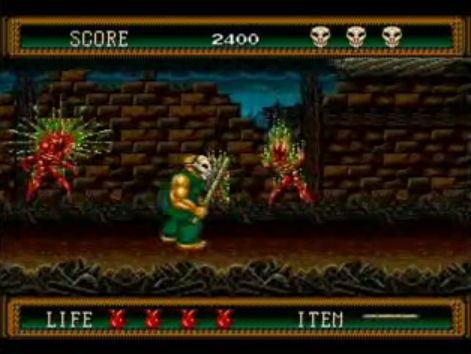In this gameplay screenshot, the top of the screen features a green banner adorned with a gold trim and bold, white text that reads "Score 2400". Additionally, there are three white skull icons displayed. Below this banner, a menacing, muscular figure with a yellow body is prominently visible. This character, reminiscent of a monster, wears a white hockey mask and is dressed in green attire while wielding a slender weapon. Flanking this central figure are two red, demon-like entities. The background reveals a partially visible stone wall in various shades of brown. The green, muscular character stands on a stretch of dirt, with a pile of bones scattered beneath them. At the bottom of the image, another green banner with gold trim is seen, which features the word "Life" in white font, next to four red objects resembling devil heads. This banner also contains the word "Item" in white font, followed by a blank white line.